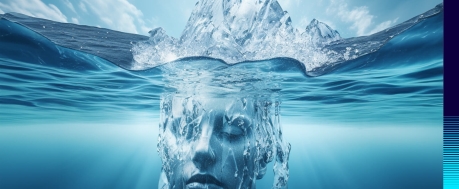The image is a computer-generated depiction of a woman's face submerged in water, captured in a horizontally aligned, rectangular frame. The scene is dominated by cool shades of blue, gray, and white. At the very top of the picture, a serene sky with blue hues intermingles softly with white clouds. Just below, a dramatic splash captures the moment the woman's head plunges underwater, creating the illusion of white waves or mountain peaks against the surface. The water's surface exhibits gentle ripples on each side of her head. Her face floats centrally within the frame; her eyes are closed, and water droplets cascade down her cheeks. Her lips mark the lower border of the image, cutting off her chin entirely. The underwater section is a gradient of dark to light blue, with darker shades accentuating the bottom corners, blending up into lighter tones directly behind her head. The surface impact is visible above her, with bubbles dotting the water around her submerged face, contributing to the sense of motion and immersion. Horizontal lines trace across the right-hand side, adding texture to the water depiction.